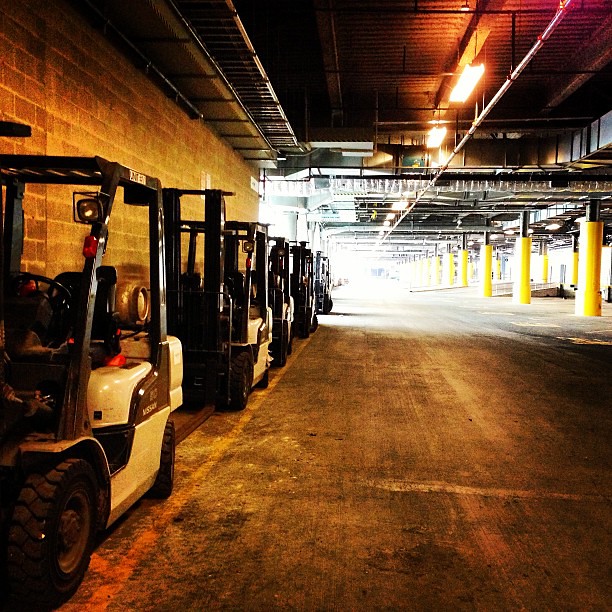This color photograph captures a spacious, warehouse-like environment with a distinctly industrial feel. The scene is set in a corridor that might be part of a manufacturing plant, a tunnel, or another large functional structure. The floor is cement, and the left-hand side features cinder block walls, while the ceiling exposes metal beams supporting long, rectangular fluorescent lights. On the right-hand side, yellow-wrapped support pillars can be seen. The most striking aspect of the image is a neat row of parked industrial vehicles, which resemble white golf carts or Kubota-type machinery, characterized by their black wheels with distinctive spokes and black canopies. The bright sunlight shining from the background obscures further details, contributing to a somewhat dystopian atmosphere. No people or text are visible in the image, emphasizing the stark, utilitarian nature of the setting.